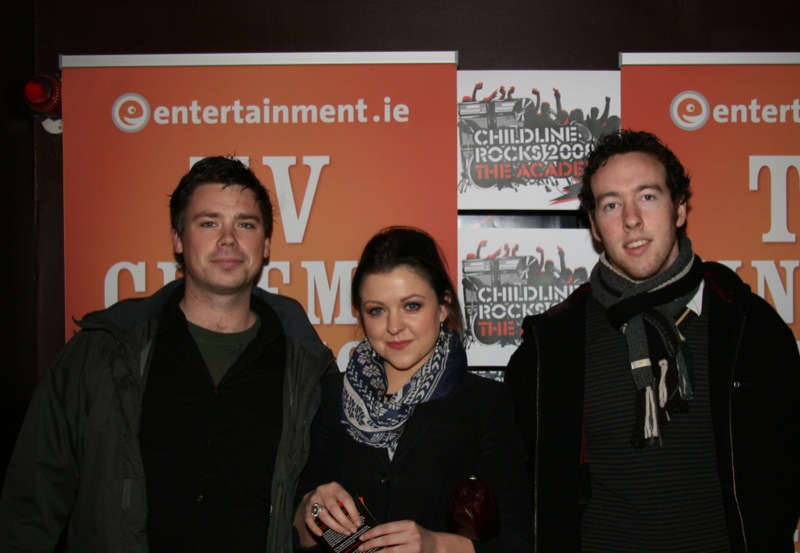The image depicts a press photograph featuring three individuals standing confidently in front of a promotional banner. Central to the background are multiple posters displaying silhouettes of people raising their fists, alongside text that reads, "Childline Rocks 2008, The Academy." Flanking these central posters are orange banners with "Entertainment.ie" written in white, accompanied by some additional unreadable text that includes "TV."

The woman in the center appears to be in her 30s, with long brown hair and light eyes, adorned with red lipstick. She is wearing a black coat and a distinctive black and white scarf around her neck. She holds a book in her hands, which are visible, showing a ring on her ring finger. On either side of her stand two men. The man on her left, who is clean-shaven with short hair, sports a black shirt under a lighter black coat. The man on her right has a bit of stubble and is dressed entirely in black, including a black coat and a scarf. The trio, dressed warmly in coats and scarves, appear to have attended a formal event or premiere, indicative of the colder environment suggested by their attire.